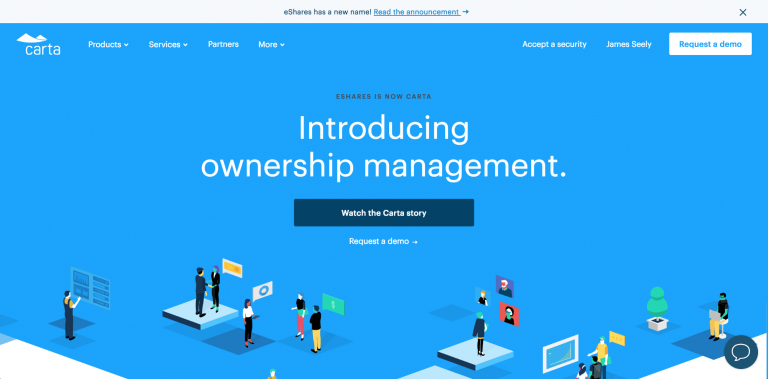This is a detailed caption for the described screenshot:

---

The screenshot features an interface from Carta, previously known as eShares. At the topmost part, there's a gray header announcing "eShares has a new name," followed by a prompt to "read the announcement" with an arrow pointing to the right and a close (X) button. Below the header, the interface features a blue background with white text.

Central to the image is what appears to be a mountain illustration situated above various menu options, including "Product," "Services," "Partners," and "More." Beneath these options, a white rectangle highlighted in blue invites the user to "Request a Demo." Just below this panel, bold dark blue text declares "eShares is now Carta," while another line introduces "ownership management."

Further down, a blue rectangle offers to let the viewer "Watch the Carta story." Inside this blue box, white text reiterates the "Request a Demo" option accompanied by a right-pointing arrow. The image also includes individuals engaging with floating, seemingly intangible computer-like technology.

In the bottom part of the screenshot, the name "James Seely" (spelled S-E-E-L-Y) is mentioned, though its context in the image is unclear.